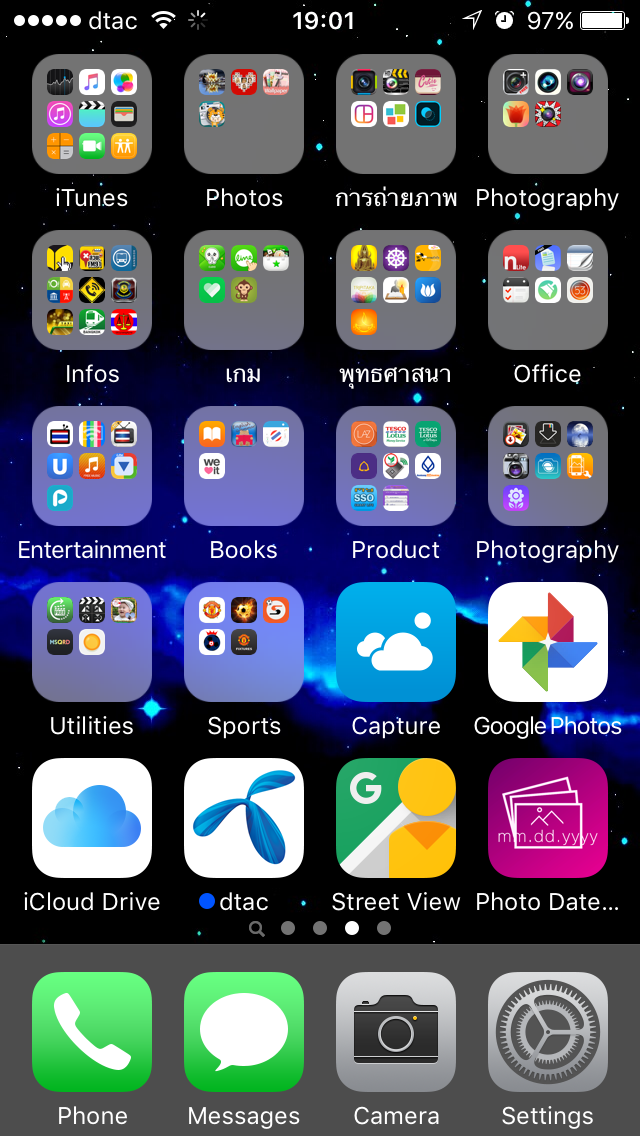The color image is a detailed screen capture of a smartphone home screen. The background of the display is black, which contrasts sharply with the various app icons arranged across the screen. There are single app icons such as "iCloud Drive," "Phone," "Messages," "Camera," "Settings," "Street View," and "Office," each with white lettering underneath in English. Some icons are grouped together, representing folders like "iTunes," "Photos," and another slightly confusing one named "Photography." Additionally, several icons or icon groups have captions written in what appears to be a South Asian script, adding a multicultural element to the display.

At the top of the phone screen, the status bar indicates a time of 19:01, suggesting that the device is set to a 24-hour clock format. The battery icon shows it is 97% charged. The top left corner of the screen reads "DTAC," potentially indicating the phone's carrier or brand, and an active Wi-Fi symbol is also visible, ensuring connectivity.